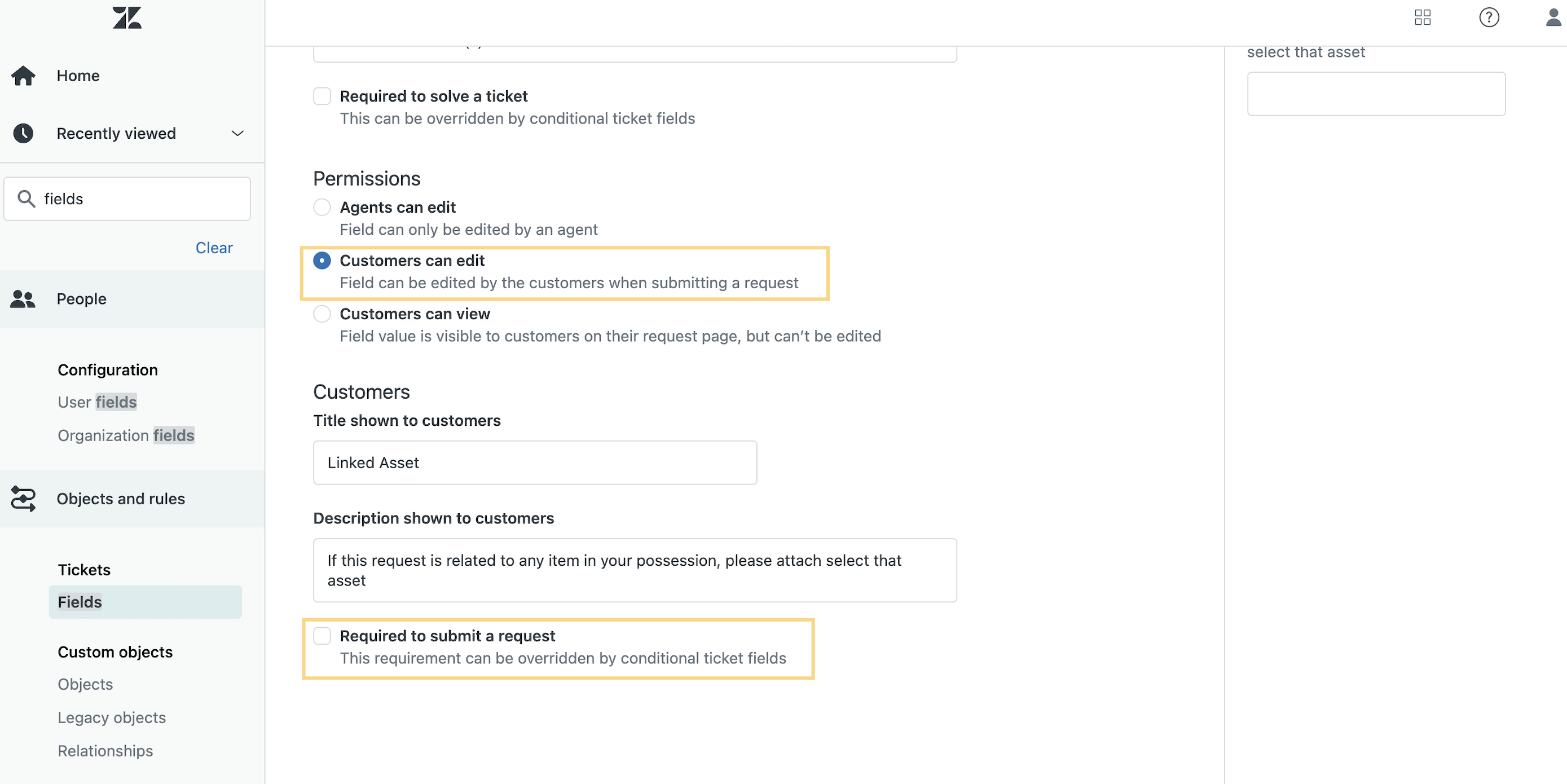This is a detailed screenshot of a website, identified by the logo containing the letter "Z". The screenshot has been digitally modified to include two prominent yellow boxes highlighting specific features of the site. The first yellow box encircles a section labeled "Customers Can Edit," prompting users to make modifications to this part of the screen. The second yellow box focuses on a section labeled "Required to Submit a Request," indicating that the user needs to fulfill certain requirements to submit a request, though the exact nature of the request remains unclear. The website interface shows that a customer is currently logged in. Several fields are present for adding customized objects or uploading user data and linked assets. Additionally, on the left-hand side, there is a text help bar to assist users with navigation and usage of the site.